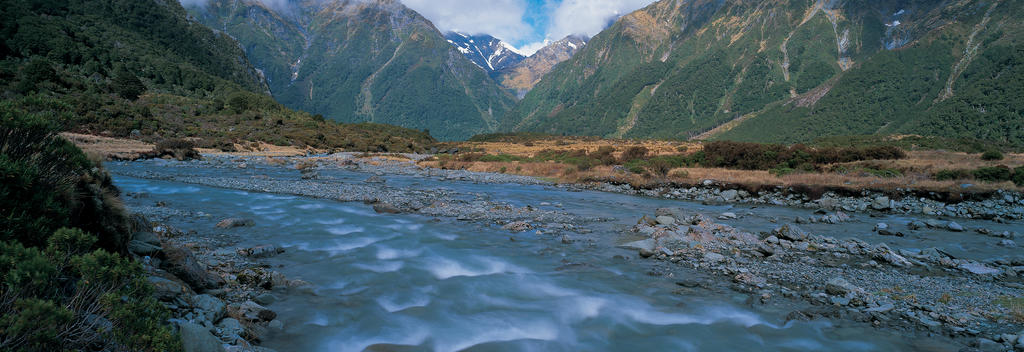The photograph captures a stunning, panoramic landscape of a shallow, fast-moving river reminiscent of those found in Alaska or the Pacific Northwest. The river, filled with exposed gray rocks, rushes swiftly, creating white-capped currents near its edges. A person, likely standing close to the bank, provides a vantage point looking down into the water, revealing the dynamic nature of the river. The left side of the image features a rocky bank in the bottom left corner, while the right bank extends horizontally across the middle of the photo, also characterized by rocks and low vegetation. Bushes and shrubs dot the edge of the river, progressively giving way to the lush, vegetated slopes of a valley. Higher up, the mountainsides become increasingly rocky and less vegetated, culminating in snow-capped peaks. Although most of the peaks are cropped out, the distant backdrop in the top middle of the photo showcases lofty, snow-covered summits under a patch of blue sky and scattered white clouds, adding depth and grandeur to the scene.